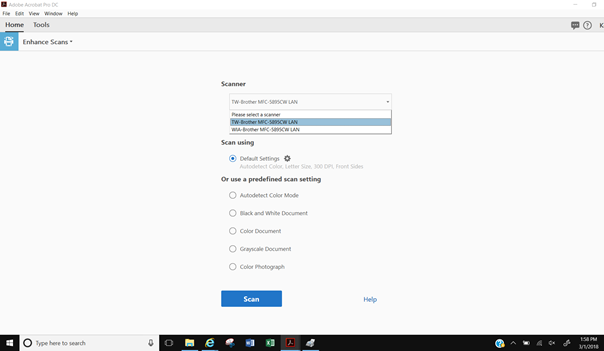The image depicts a screenshot of the Adobe Acrobat DC interface. The top section features a blurry white background with faint gray text indicating "Adobe Acrobat DC." Below this are the main menu options in black text: "File," "Edit," "View," "Window," and "Help." Underneath, the interface transitions to a gray background featuring the labeled sections "Home" and "Board," along with an underlined "Tools" section.

On the right side of the image, a gray text box displays eight circular icons. One of these icons is a gray-outlined circle with a white interior and a gray question mark inside. Adjacent to this, an incomplete word beginning with "K" is visible, though the rest is cut off.

Further down, there's a blue box with a white printer icon, next to which is black text that reads "Enhance Scans" and "Scanner." The scanner section includes a scroll box with selectable options, showing the end of a selection labeled "L-E-N."

Highlighted in blue, a selection box shows the prompt "Scan Using" with the "Default Settings" option selected, indicated by a blue-filled circle. Additional options listed are "Auto Detect Color Mode," "Black and White Document," "Color Document," "Gray Scale Document," and "Color Photograph."

At the bottom, there is a blue button labeled "Scan" in white text, and to its right, another option labeled "Help" in blue.

This detailed breakdown outlines the interface elements present in the Adobe Acrobat DC screenshot.